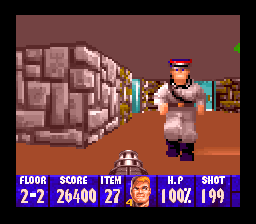A detailed and cleaned-up description of the image could be:

"This image is a screenshot from a video game, presented in a square format with a thick black border surrounding it. At the bottom of the image, there is a series of blue panels displaying various gameplay metrics. These panels feature light white and yellowish text indicating 'Floor,' 'Score,' 'Item,' 'HP,' and 'Shot,' with corresponding numerical values beneath each label. In the central panel, a character's face is prominently displayed; the character has orange hair, light skin, and a stout expression. The main in-game scene shows a solid brown floor with a gun visible from a first-person perspective, pointing forward. The background consists of stone and brick walls, and a person dressed as a military officer is seen walking towards the camera."